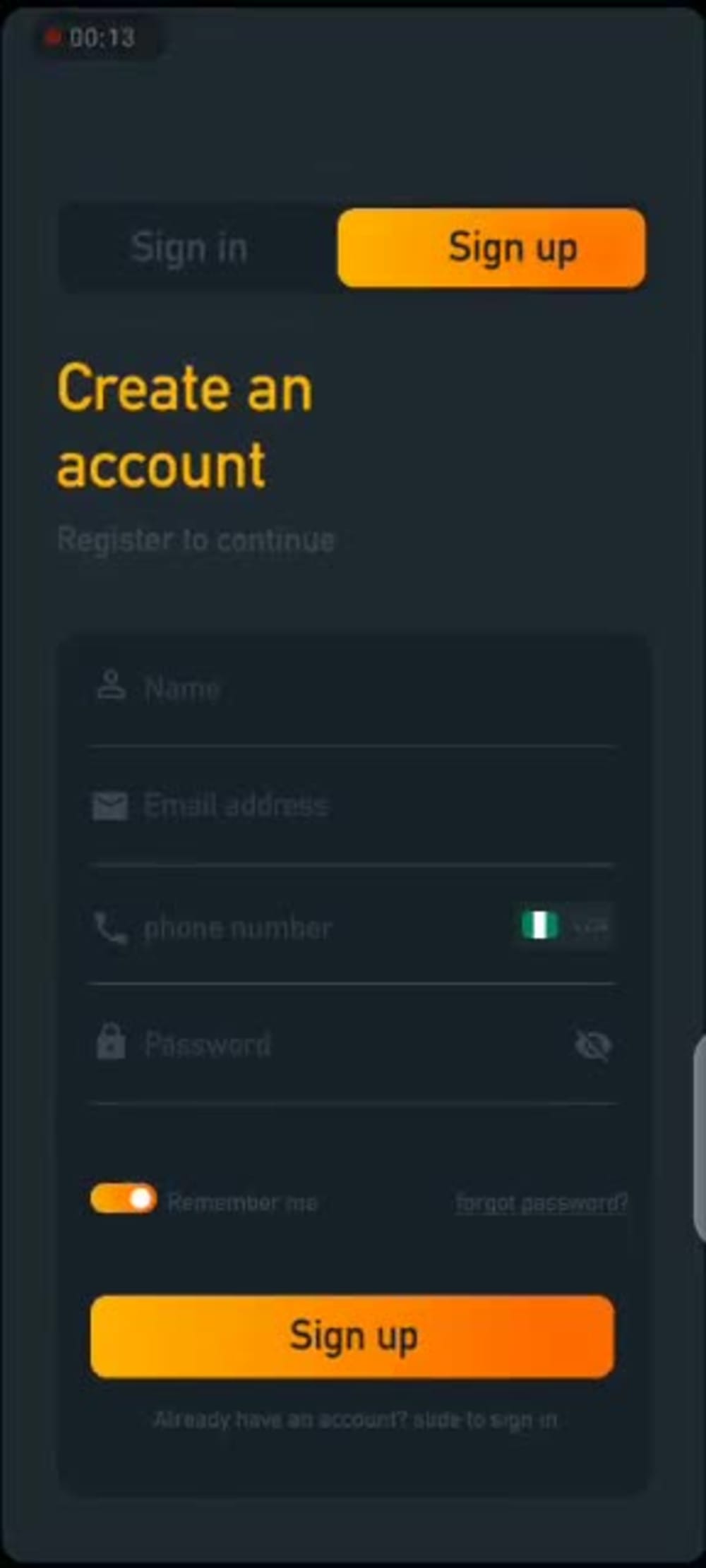This image showcases a user interface screenshot from a registration page. At the top, there is a small red notification dot accompanied by the number "013." Below this, there are buttons labeled "Sign In" and "Sign Up," with the latter being a prominent yellow-orange button. 

The page instructs users to create an account, featuring the text "Create an Account" in yellow. Below this, there is a message that reads "Register to Continue, Integrate." An interactive form follows, allowing users to input their details. This form includes fields for name, email, phone number (with a Nigerian flag icon suggesting Nigerian usage), and password. Each field is accompanied by relevant icons, such as a person icon for name and a phone icon for the phone number. 

An "Remember Me" checkbox is highlighted in orange, and there's also a "Forgot Password" link for users who need to reset their passwords. The "Sign Up" button is also orange with black text. 

The background of this application is dark, appearing either black or very dark blue. At the bottom of the page, there's a prompt for users who already have an account, asking "Already have an account?" with an instruction to "slide to sign in." There's also a "Sign In" button at the top for returning users.

The overall design suggests that this is a registration interface, although the specific service it pertains to is not clear from the screenshot alone.